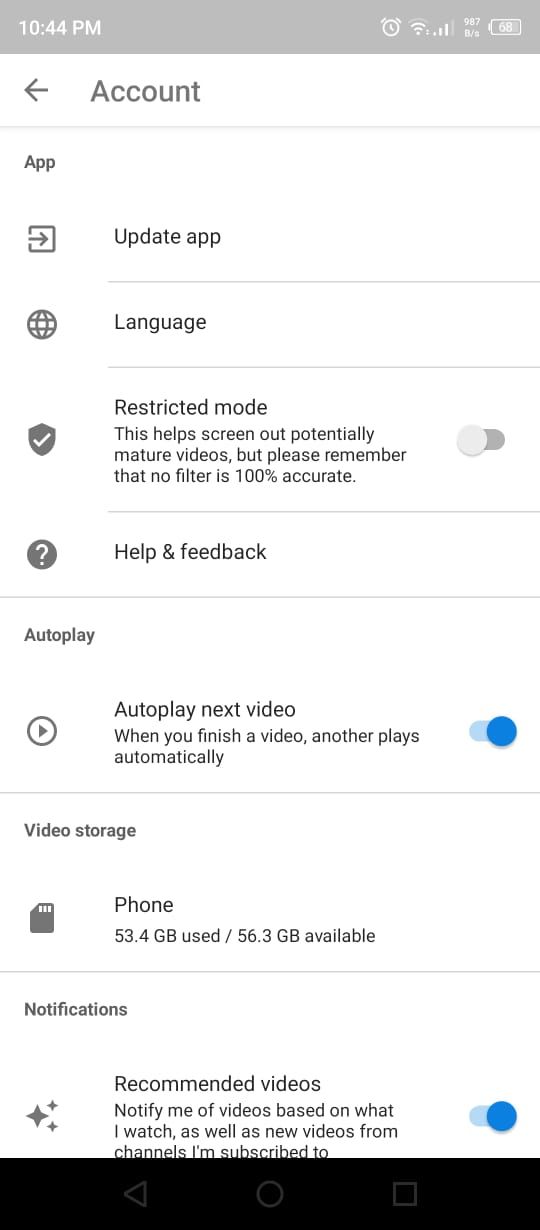The image displays a cell phone screen showcasing the account settings menu. At the top left of the screen, the time is indicated as 10:44 PM. On the top right, there are three icons: one for Wi-Fi, one for cellular connection, and one for battery percentage.

The main section of the screen is titled "Account." Underneath this title, there are several options listed:

1. **App**
2. **Update App**
3. **Language**
4. **Restricted Mode** (which is set to off)
5. **Health and Feedback**

Following these primary options, another section starts with "Auto Play." Here, the option "Auto Play Next Video" is toggled on, as indicated by a blue button pushed to the right.

Further down, there's a section for "Video Storage," showing that the phone has 53.4 GB used and 56.3 GB available.

Another option listed is "Recommended Videos," which is also toggled on, signified by a blue button pushed to the right.

At the very bottom of the screen, the background turns black and features three navigation buttons. On the left is a sideways triangle (likely a back button), in the middle is a circle (possibly the home button), and on the right is a square (potentially the recent apps button).